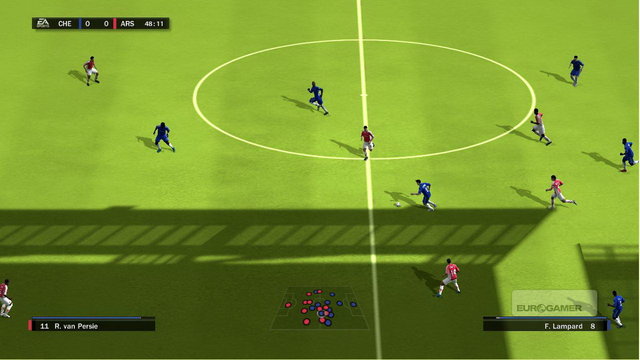In this still shot from a soccer video game, an aerial perspective captures an expansive view of a vibrant green field marked with traditional lime-colored soccer lines and the central circle bisected by the halfway line. On the field, two teams—one in red and the other in blue—comprising around 11 to 12 players each, are actively running around. The digitally-rendered game environment features interactive elements, including a square near the front of the image showing red and blue dots representing player positions. On the right side of the screen, a digital nameplate displays "F Lombard 8," with "Eurogamer" above it, possibly the name of the game or a related entity. Another nameplate on the left reads "11 R Van," with the rest of the name obscured. The top-left corner presents the scoreline, with "CAG" versus "ARS" at 0-0 and a timestamp of 48 minutes and 11 seconds into the game.